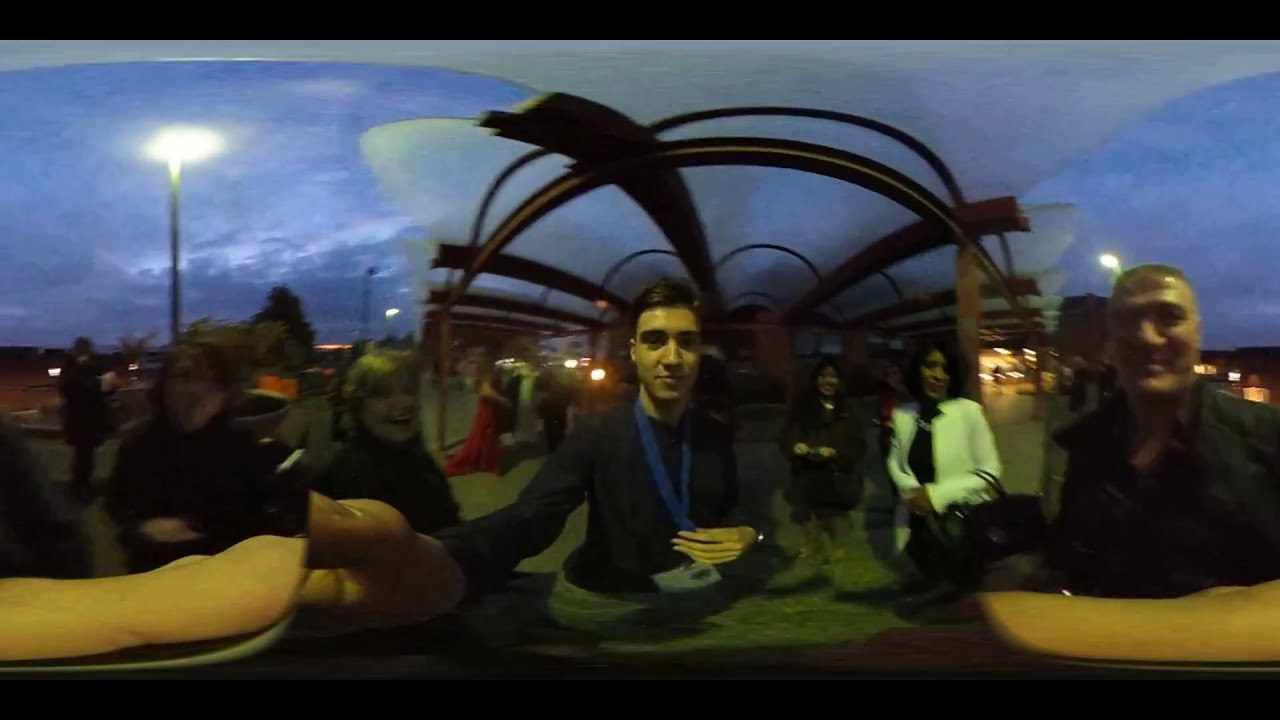This image, taken outside in the early evening, captures a bustling, lively scene where people are gathered around what appears to be a public event or an outdoor counter, possibly for food. The photograph is horizontally rectangular, with thin black stripes framing the top and bottom, and is slightly widened to the point of blurriness. The sky is a dark blue with some overcast gray clouds, and streetlights illuminate the scene, creating a softly lit atmosphere as twilight descends.

At the center of the image stands a clean-shaven man with short hair, wearing a black jacket over a blue shirt, and a blue lanyard with an ID card around his neck. His hand, possibly reaching for some food, rests on a gray plate with brown bread on the counter. To his left, a smiling woman in a dark jacket gazes into the camera. On his right, three individuals stand close by: a woman in black with a gold necklace, another woman in a black shirt and white blazer, and an older man in a dark-colored, long-sleeved collared shirt who also looks directly into the camera.

The overall scene is one of interaction and camaraderie, with people smiling, laughing, and talking, creating a vivid tableau of social engagement against the softly lit, early evening sky.